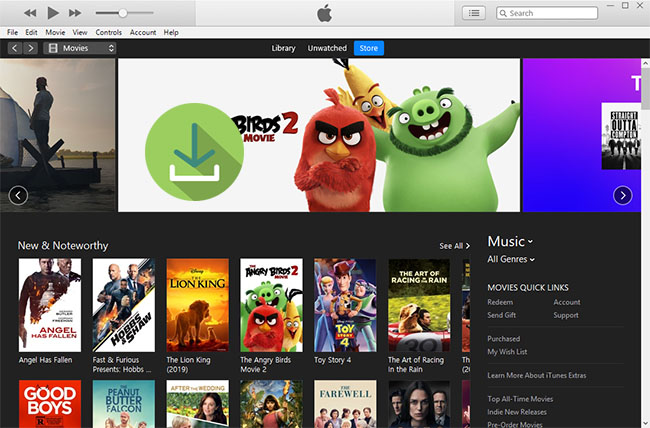The image showcases a screen from a Mac product, unmistakable due to the Apple logo centered at the top. To the left of the logo are the video control buttons, while a search bar occupies the right side. The topmost section of the display includes menu options such as File, Edit, Movie, View, Account, and Help. Dominating the center of the screen is a visual display for the animated movie "Angry Birds 2," alongside an indication for download availability.

On the left side of the screen, there's an image of a man standing on a raft in the middle of a body of water, adding a contrasting visual element. To the right, another prominent display features the movie "Straight Outta Compton." Below this primary content area, the screen lists "New and Noteworthy" movies, flanked by a section dedicated to "Music - All Genres." Further down, quick links are provided, including categories like "Movie Quick Links," "What's Been Purchased," "My Wish List," and "Learn More About iTunes Extras."

Additional sections highlight "Top All-Time Movies," "Indie New Releases," and "Pre-Order Movies." The genres of the showcased movies range widely, representing a broad spectrum of tastes and interests. The overall layout underscores a diverse and rich array of entertainment options available on the platform.